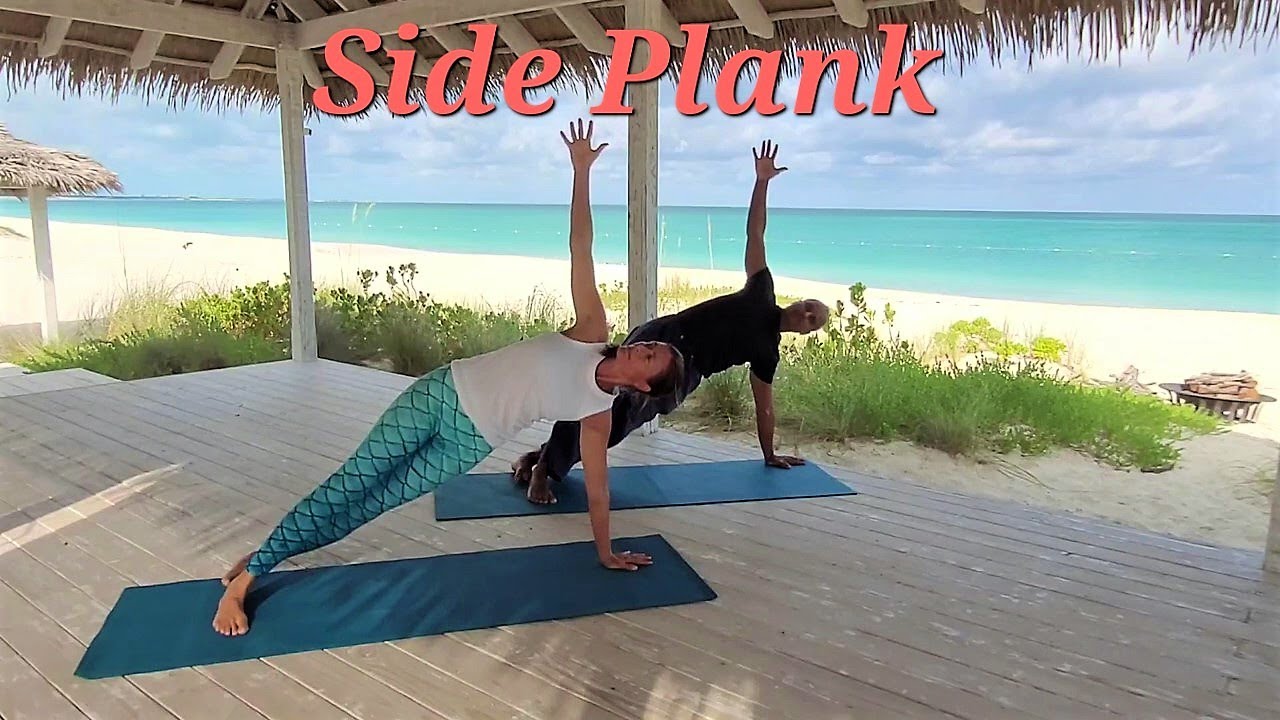In this vibrant tropical setting, two individuals practice yoga on blue mats under a wooden canopy with a thatched roof. The scene is set against a backdrop of a light blue sky with wispy white clouds and pristine turquoise water. The sandy beach is visible beyond the structure, and light green plants with yellow flowers add to the lush ambiance. In the foreground, a woman in a sleeveless white tank top and blue leggings with a darker blue cross-hatching pattern holds a side plank position. Behind her, a man dressed in a black top and sweatpants mirrors the same yoga pose. The top of the photograph is marked with the words "SIDE PLANK" in large pink letters, suggesting that this image may be part of an instructional guide.